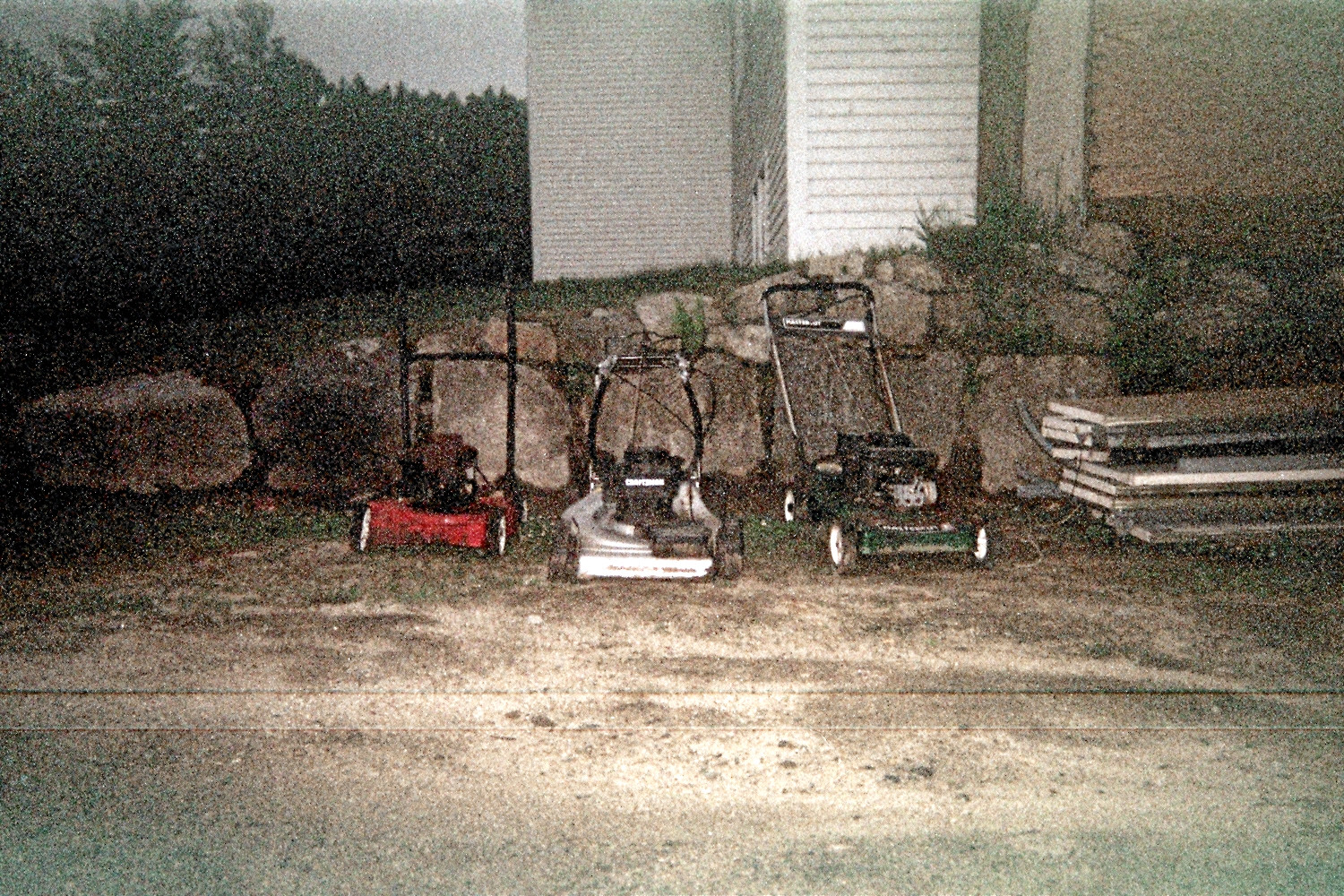In this grainy, landscape-oriented photograph, likely taken with a 35mm film camera from the 1990s using a flash, the scene captures an outdoor setting in low light. Central to the image are three petrol lawnmowers positioned on a patch of dirt and dead grass, directly in front of a large boulder retaining wall. From left to right, the lawnmowers are red, white, and green, each with varying handle heights. Behind them, a stack of door-sized wooden planks is visible to the right. In the background, partially obscured by the retaining wall, stands a weatherboard house with a visible tree trunk nearby. Further to the left, a dense cluster of trees and grass can be seen, suggesting a wooded area beyond the house.